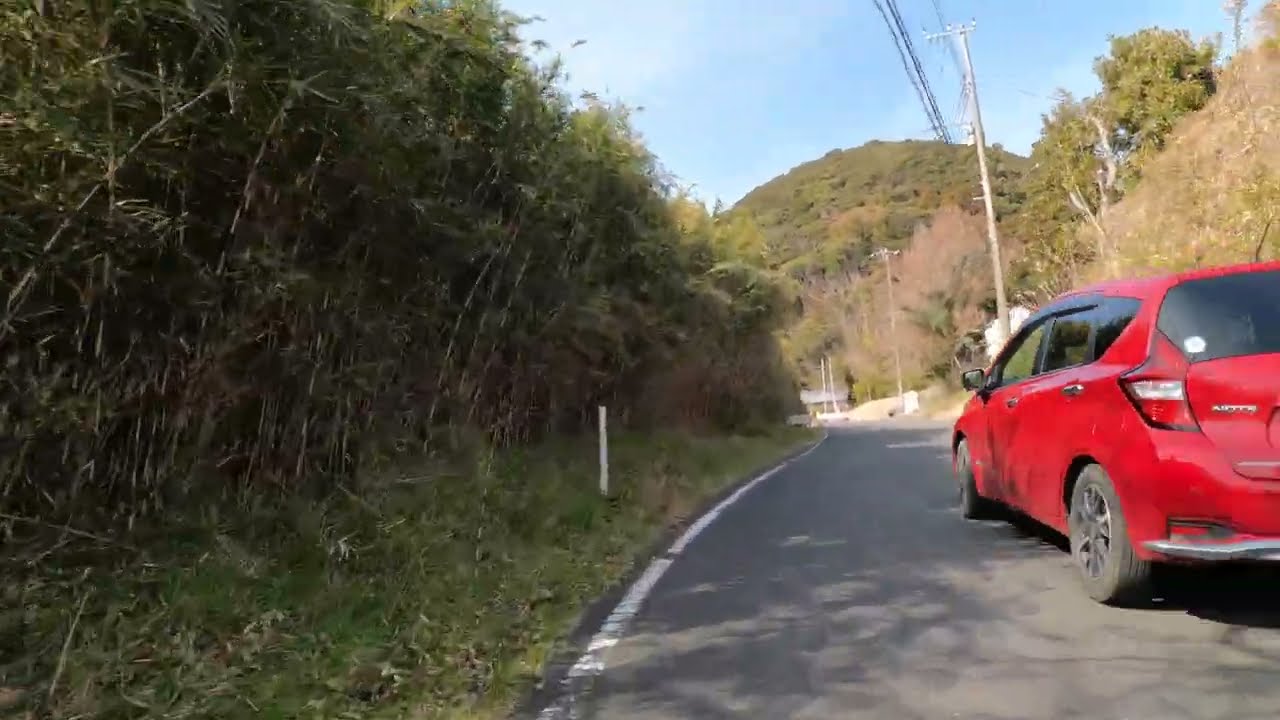This outdoor daytime photograph features a narrow, curved paved road that winds between two green hills. The road occupies the right half of the image, while tall, bamboo-like plants and thick greenery dominate the left. A red, four-door hatchback, likely a Ford, is prominently displayed, with its back end facing the viewer and partially cut off by the photo's edge. Above, power lines stretch across the blue sky, dotted with a few clouds. To the right, a telephone pole stands tall. The distant hillside is lush with short green trees, contrasting with a single dead tree visible on the right side of the road. The vivid colors of the scene include the red of the car, the gray of the asphalt, the rich greens of the vegetation, and the bright blue of the sky, all captured in a realistic, representational style.